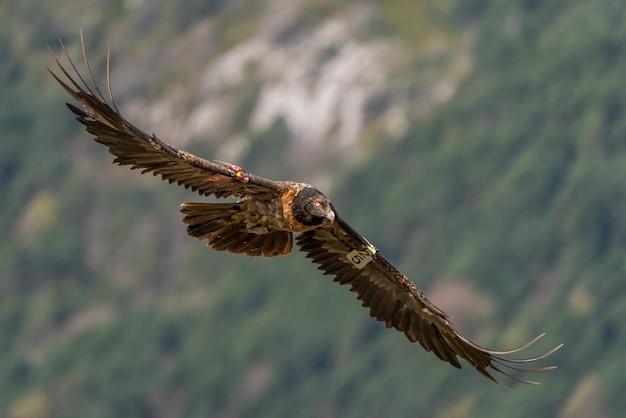This image captures a majestic bird, likely a hawk or falcon, in mid-flight. The bird's impressive wingspan extends diagonally from the top left corner to the bottom right corner of the frame. It has its wings fully spread, showcasing a rich array of feathers, with five prominent ones visible at the tips. The bird's head is more arrow-shaped, featuring a sharp white beak and a darker brown coloration on its face and neck. A beige tag marked with the number 25, displayed vertically, is attached to its left wing (on the right side of the image), and there may also be another unidentified tag on its right wing. The background is an out-of-focus blend of greenery and a blurred mountain range, emphasizing the bird as the central subject of this dynamic action shot.